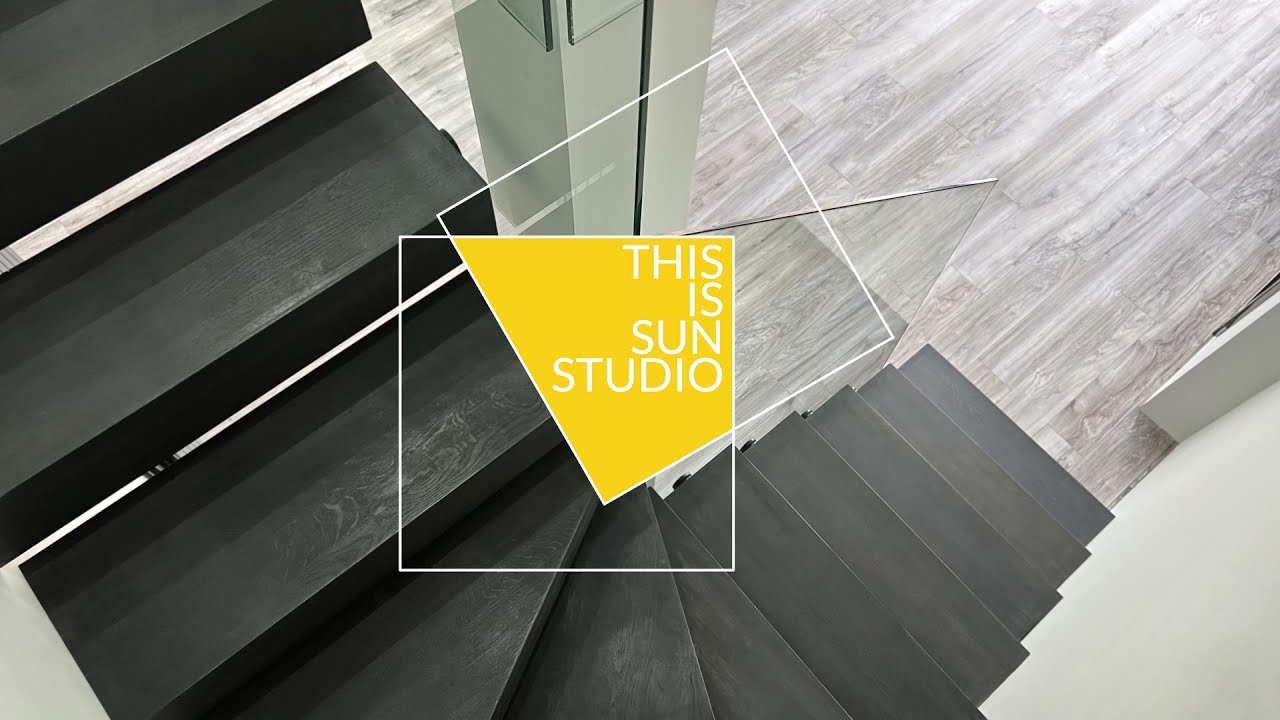The image portrays a stylized, graphic art advertisement featuring a twisting staircase. From an elevated viewpoint, likely the second floor, the black wooden steps descend diagonally from the left to the center of the image before making a 90-degree turn and continuing upward toward the top right. The stairs appear mid-image, framed by tan walls and a floor made of light beige wood, interspersed with darker beige tones. Centrally superimposed are two offset white-outlined squares, overlapping to form a yellow area that reads "This is Sun Studio" in white letters. Above this focal point, a support pillar divides the stairwell, adding structural context to the visually engaging composition. The photograph serves as an advertisement, blending intricate architectural features with clean, modern graphic design elements to highlight the studio's identity.